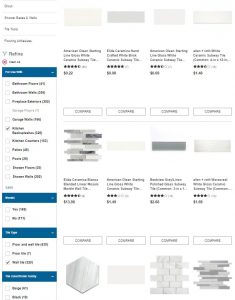**Caption:**

The image depicts a series of small, illegible text boxes arranged in a grid format. On the left side, there is a sequence of text boxes alternating in colors: starting with white text on a black background (completely unreadable), followed by blue text on white, then several black text boxes, another blue on white, two more in black, one in white, three in black, and finishing with blue on white and two in black once again. 

On the right side, there are four crossed sections, each showcasing images of various objects accompanied by black text with pricing details. Due to the small size and poor resolution of the image, the text remains unreadable. The objects depicted resemble high-end kitchen or bathroom tiles—possibly ornate glass tiles with gray-on-gray designs. Unfortunately, the diminutive size and low-quality font render further details indistinguishable.